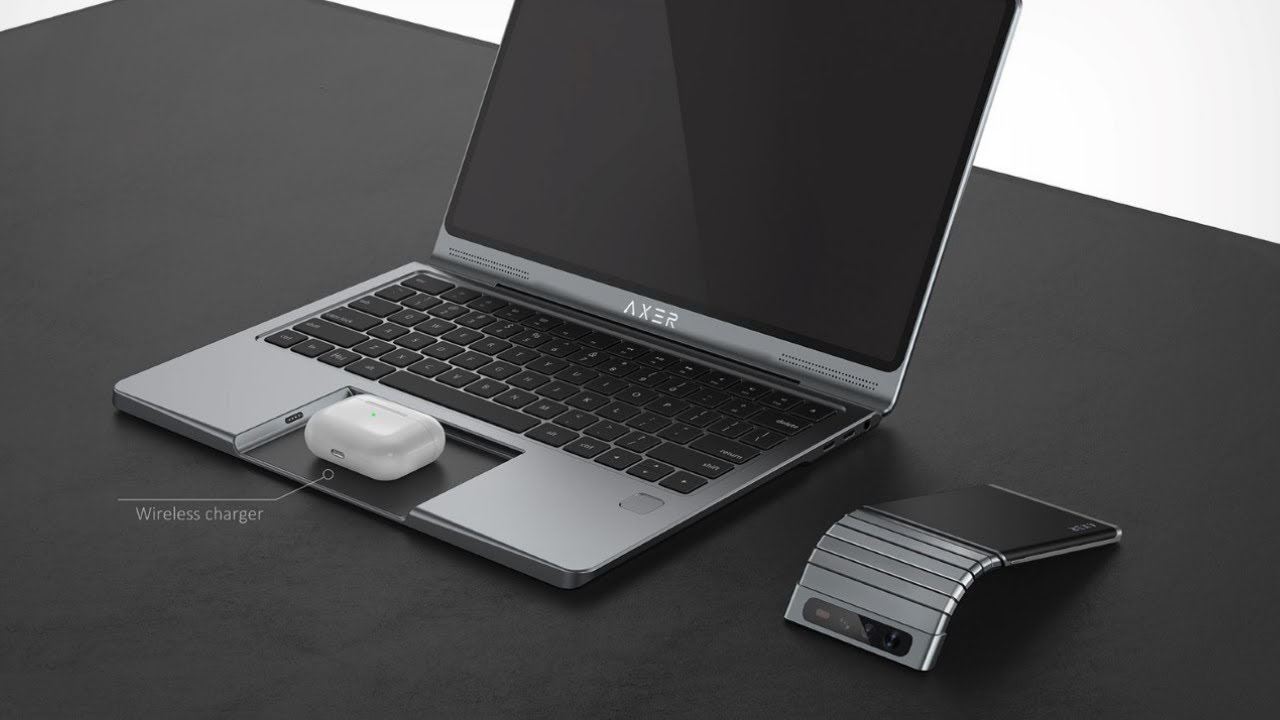This color photograph showcases a sleek silver laptop, branded with "Exer" below the screen, resting diagonally on a black table against a neutral white-gray background. The laptop's screen is turned off, and it features a standard black keyboard. Instead of a traditional trackpad, there's a rounded rectangle-shaped wireless charger occupying the space, characterized by a blue light on top and a front-facing USB port. Next to the laptop, a raised and adjustable trackpad is positioned, elevated slightly by a flexible metal joint. The minimalist setup highlights the innovative design, perfect for a tech advertisement.